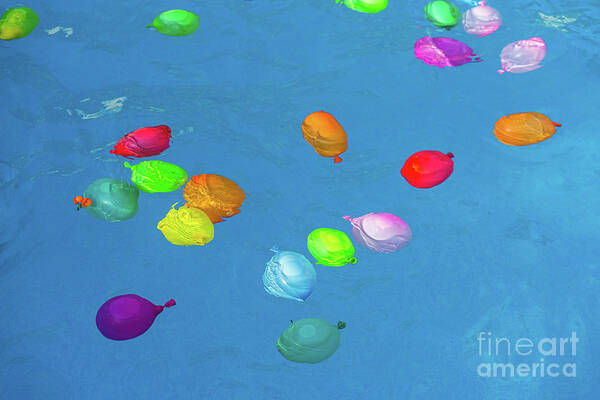The image features a vibrant and whimsical scene that appears to be a painting and could be interpreted either as balloons in water or the sky. It presents a solid blue background, subtly textured with shades of white and gray to suggest delicate ripples or clouds. Scattered across this background are numerous colorful, oval-shaped objects resembling deflated balloons or fish with small ties at their ends. These objects are arranged predominantly in clusters, with green ones starting at the upper left corner followed by a mix of purple, pink, red, orange, and yellow hues spread across the scene. The middle section features a prominent cluster with a red balloon beneath a green one flanked by orange balloons. Towards the lower left, there are additional colorful balloons, including purple, blue-green, and gray. In the lower right-hand corner of the image, the words "fine art" and "America" are inscribed in a subtle white font.